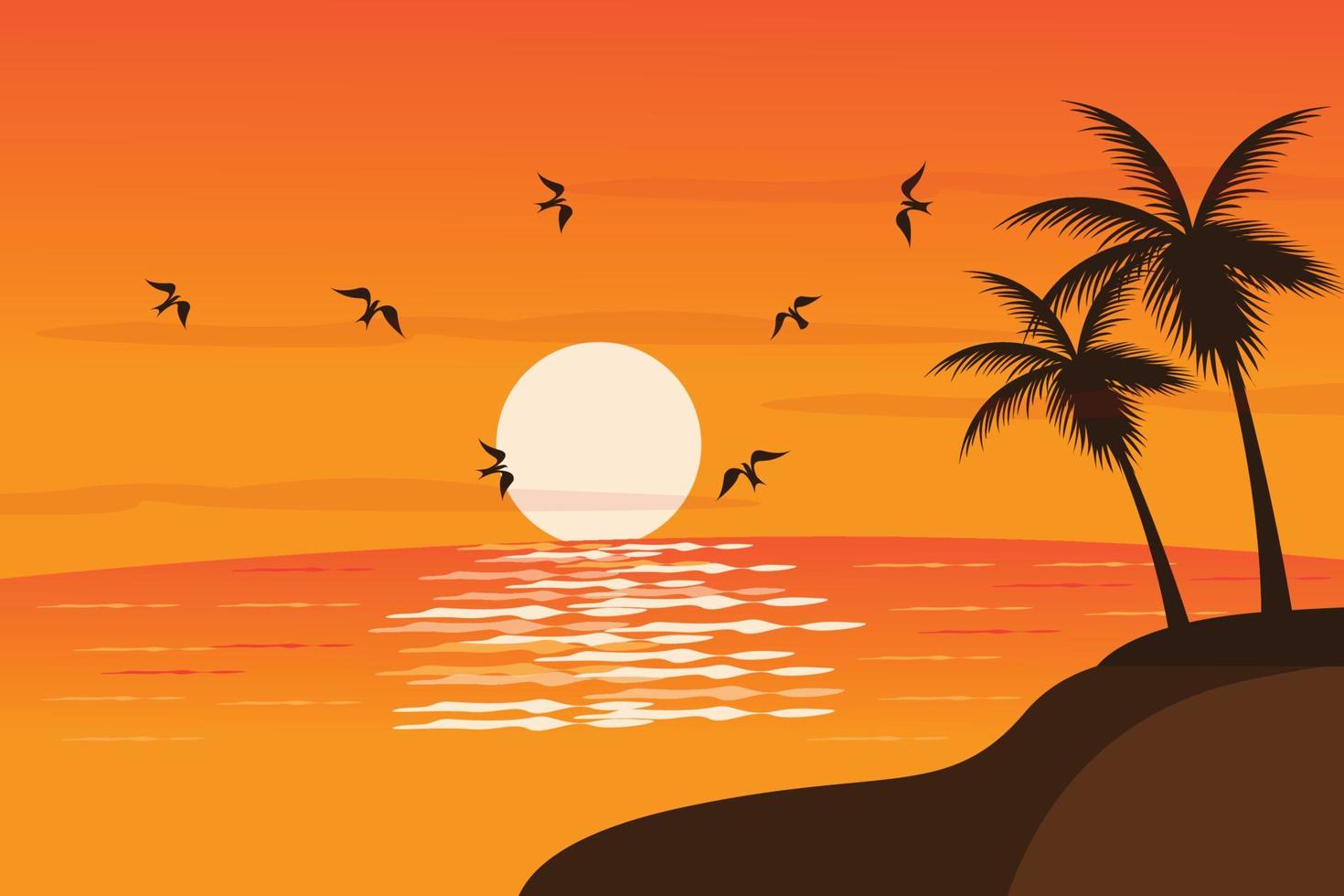The image resembles a vintage postcard with a predominantly orange background. Dominating the center is a yellowish-white circle representing the sun, casting its bright reflection on the water below, where white patches glimmer on the surface. The scene is serene, silhouetted birds, likely seagulls, glide effortlessly across the sky and in front of the sun. On the lower right, an island emerges, featuring a landmass in shades of dark brown to lighter brown. Two tall palm trees rise from this island, their spiky leaves and trunks also appearing as dark silhouettes. Horizontal clouds stretch across the sky, adding depth to the atmospheric backdrop. The entire composition exudes a warm, tranquil ambiance, capturing the serene interplay between sky, sea, and nature.